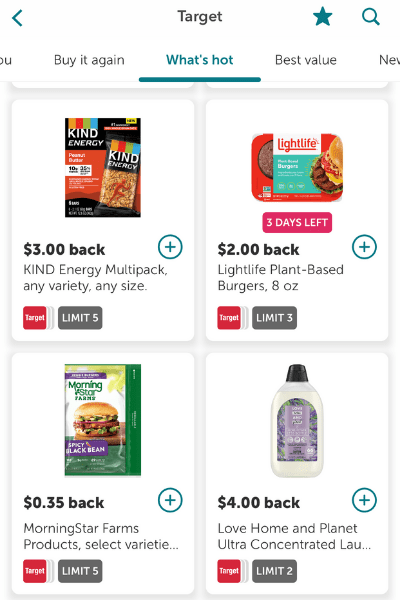This image is a screenshot from the Target app or website interface. At the top of the screen, the Target logo is prominently displayed with a blue star to its right and a magnifying glass search icon. Below the logo, navigation options are listed: "Buy Again," "What's Hot," "Best Value," and "ME," suggesting a section for new items. The "What's Hot" option is selected and underlined.

The main section of the screen shows four promotional offers arranged in a 2x2 grid. 

**First Column, First Row:**  
- *Kind Energy Bars*  
- Promotion: $3 back  
- Description: Kind Energy Multipack, any variety, any size  
- Additional Info: Limit of 5  
- Buttons: A gray button labeled "Limit 5" and a blue plus sign for adding the item to the cart

**Second Column, First Row:**  
- *Light Life Plant-Based Burgers*  
- Promotion: $2 back  
- Description: Light Life Plant-Based Burgers, 8 oz  
- Additional Info: Limit of 3  
- Urgency Indicator: "3 days left" in red text  
- Buttons: A plus sign for adding the item to the cart

**First Column, Second Row:**  
- *MorningStar Farms Burgers*  
- Promotion: $0.35 back  
- Description: MorningStar Farms Products, selected varieties  
- Additional Info: Limit of 5  
- Buttons: A plus sign for adding the item to the cart

**Second Column, Second Row:**  
- *Love Home and Planet Ultra Concentrated Laundry Detergent*  
- Promotion: $4 back  
- Description: Ultra Concentrated Laundry Detergent  
- Additional Info: Limit of 2  
- Buttons: A plus sign for adding the item to the cart

Each product image is accompanied by a description of the offer and a limit on how many times the promotion can be redeemed.